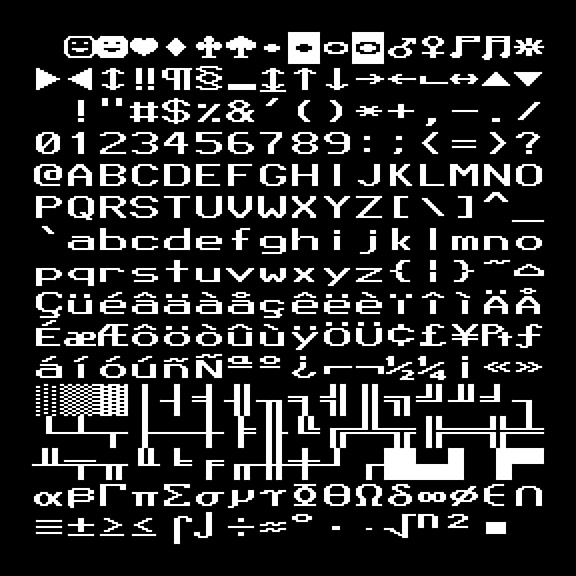The image features a solid black background filled with an array of diverse symbols and characters, seemingly arranged in distinct rows. The first row showcases various smiley faces, a heart, a diamond, a tree, a spade, a plus sign, another plus sign, two circles, male and female symbols, two music notes, and a star. Below that, a second row contains triangles, arrows pointing in different directions, exclamation points, and other unfamiliar symbols.

The third row is composed of common punctuation marks: exclamation point, quotation marks, hashtag, dollar sign, parentheses, ampersand, more parentheses, stars, plus sign, comma, dash, period, and a diagonal line. The fourth row displays the numbers 0 through 9 in sequence, followed by ellipses, a semicolon, brackets, an equal sign, and a question mark.

Descending further, the fifth row begins with an at symbol (@), followed by two rows showcasing the English alphabet in capital letters from A to Z. The capitalized letters are neatly arranged with brackets at the row's end. The next two rows display the alphabet in lowercase, from a to z, also in correct order, ending with sweeping lines.

The subsequent three rows are populated with a variety of symbols from other languages, featuring numerous accents placed above and below the characters. These lines give a multicultural and linguistic flair to the composition. At the very bottom, there is a maze-like pattern made up of double lines, twisting and turning in different directions, adding an intricate and complex finish to the overall design.